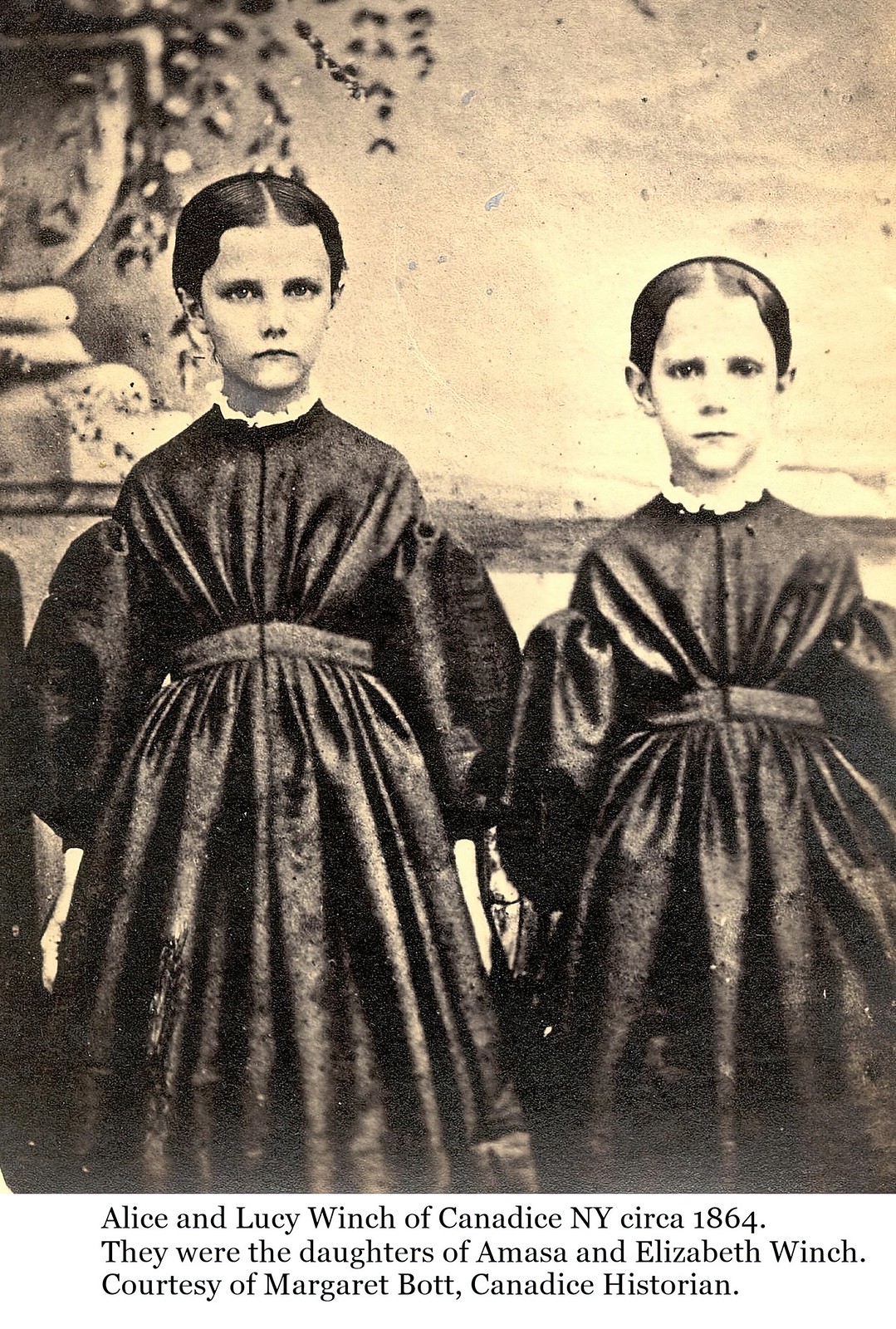This incredibly old, sepia-toned photograph from circa 1864 features two young girls, Alice and Lucy Winch of Canadis, New York. Both girls have dark hair parted exactly in the middle, pulled back tight, and exhibit expressionless or slightly angry faces. They are dressed identically in long, dark-colored dresses with lace around the neck, cinched waists, and voluminous sleeves billowing out. The skirts of their dresses are extremely full and tightly pleated. They stand in front of a backdrop that seems to depict a painted landscape, which includes a field or ocean and foliage in a planter in the top left-hand corner. Text beneath the photograph identifies them as the daughters of Amasa and Elizabeth Winch, with the preservation of this image credited to Margaret Bott, the historian of Canadis.